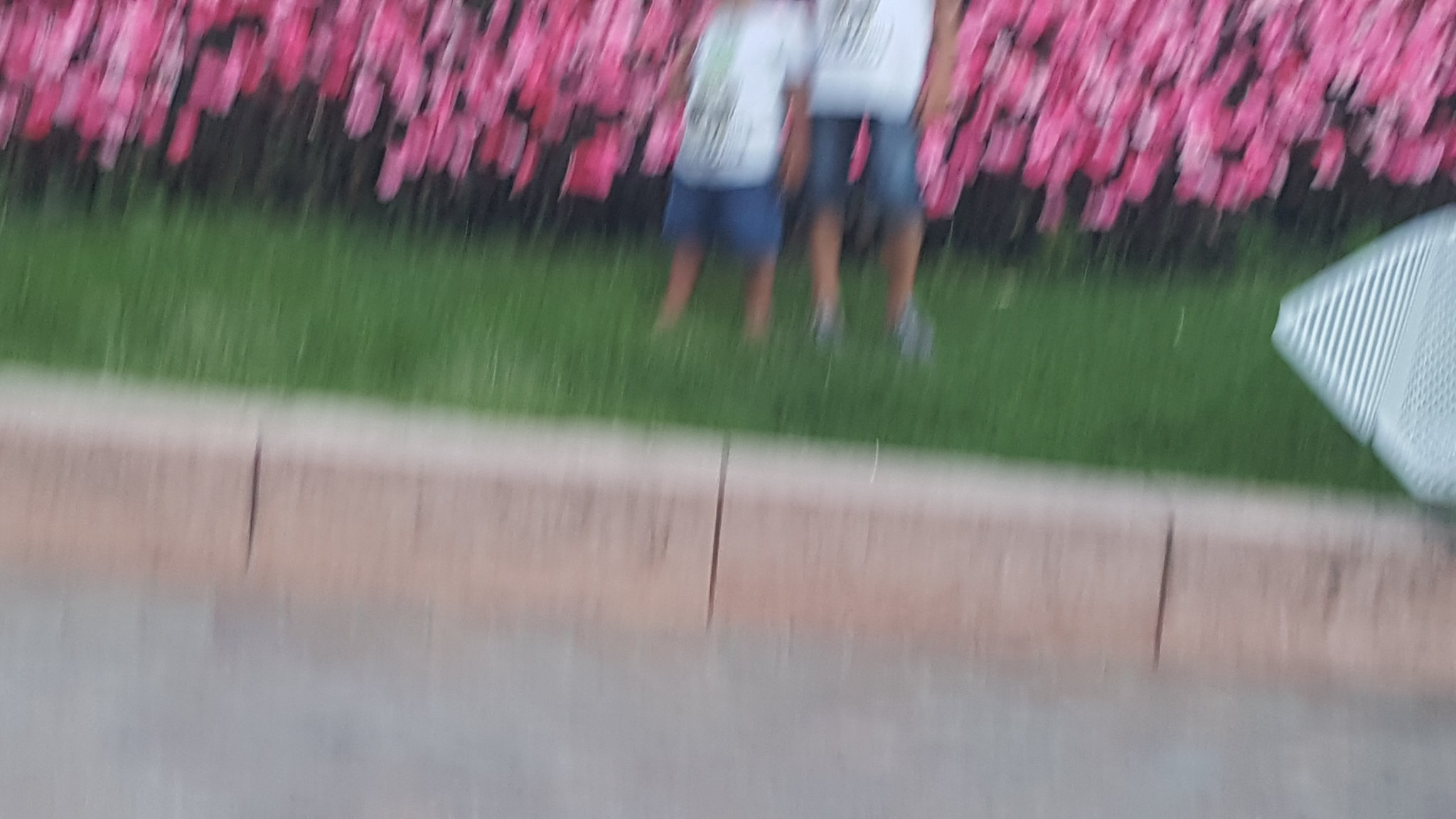In this blurry horizontal color snapshot photograph taken outside, two children stand in front of a vibrant backdrop of pink flowers and greenery. The children, positioned behind a light beige cement curb on a grassy field, have their heads cut off at the shoulders due to the framing, highlighting their torsos and legs instead. They wear matching outfits consisting of white T-shirts, possibly adorned with a Mickey Mouse logo, and blue jean shorts. A blurred road lies in front of the curb. The photograph features an artistic blur, suggesting the camera moved vertically during the shot, accentuating the pink flowers above and casting shadows from the garden below. On the right side of the image, there is an indistinct striped or wicker-like object. The overall impression is of a bright day with slightly overcast skies.